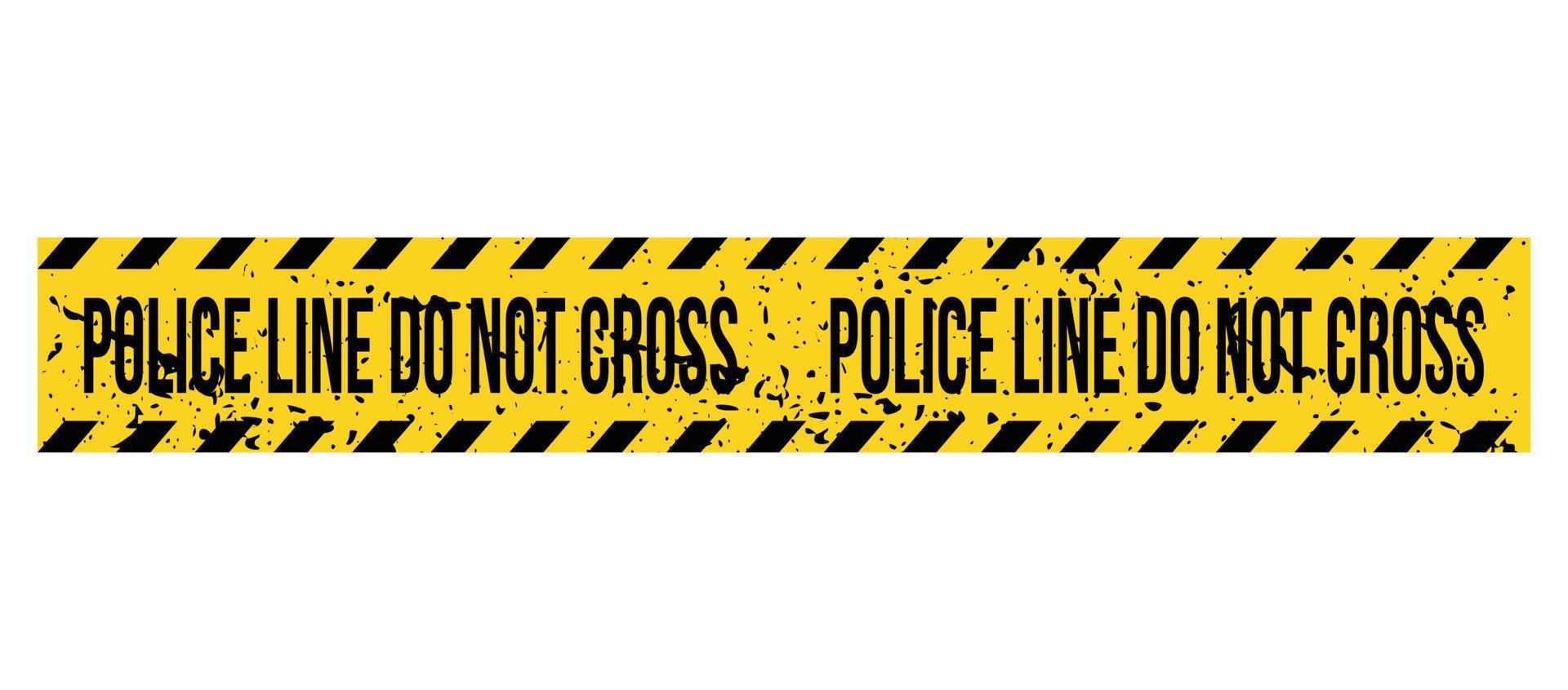The image depicts a yellow police caution tape commonly used to cordon off crime scenes and prevent tampering with evidence. The tape, approximately three and a half inches wide, prominently features black lettering that reads "POLICE LINE DO NOT CROSS," which repeats along its length. Along the edges of the tape, there is a distinct slanted square pattern. Notably, this particular strip is marked with black speckles, possibly paint, indicating prior use. The entire scene is set against a stark white background, emphasizing the tape's bright, school bus yellow color and the repetitive cautionary message. This tape is a familiar sight both in real-life crime scenes and as a decorative or prop item in stores.